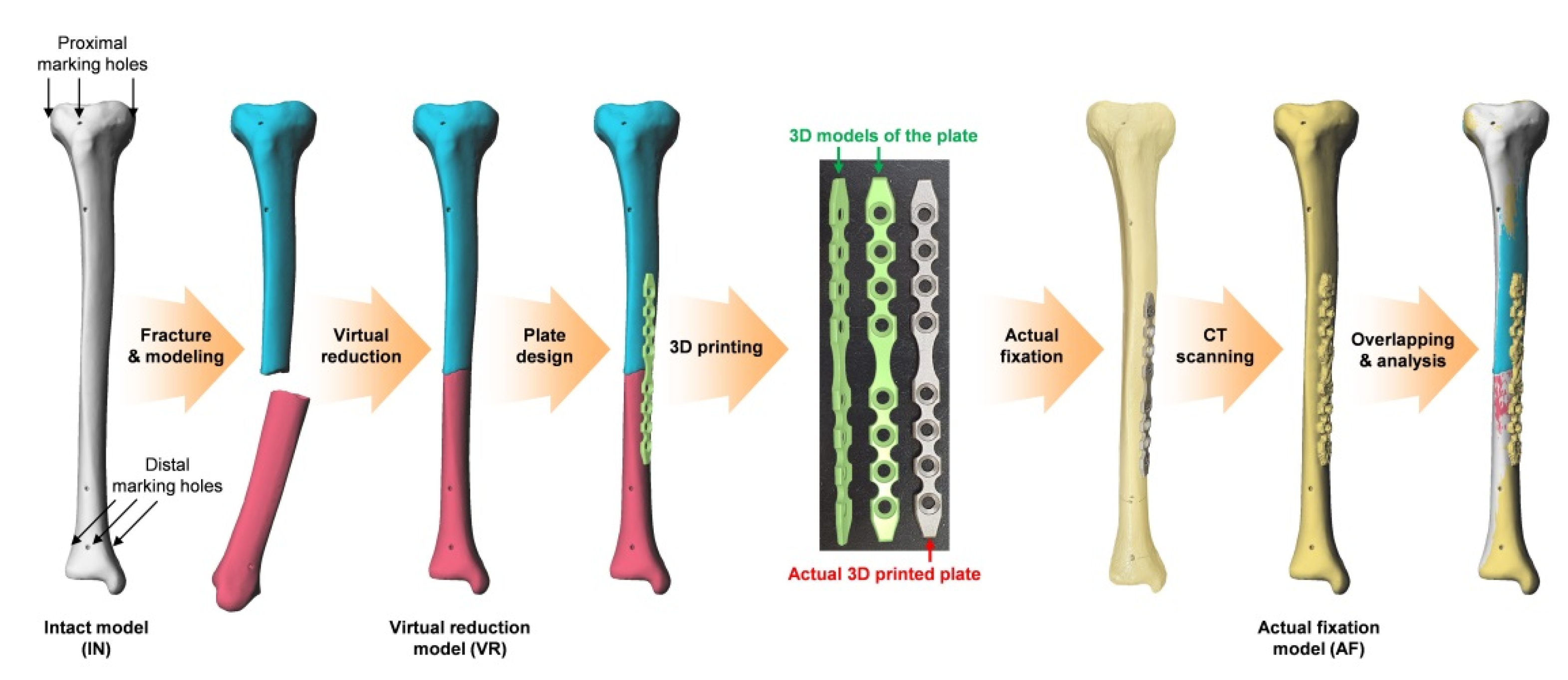The image displays a detailed medical chart illustrating the process of fixing a femur bone fracture. On the left, a plain white bone is labeled "Intact Model" with arrows pointing to three spots, labeled "Proximal Marking Holes." Next to it, a fractured bone, colored blue at the top and pink at the bottom, is labeled "Fracture and Modeling." Further to the right, the bone is shown repositioned with the tag "Virtual Reduction," followed by the "Plate Design" phase where a green chain-like plate is depicted connecting the broken segments. This is succeeded by a section on "3D Printing," showcasing three different versions of the printed plates. To the far right, three bones in varying shades—pale tan, darker tan, and a multi-colored bone—illustrate the "Actual Fixation" using the plate. Additional annotations include "CT Scanning," "Overlapping Analysis," and further hints of advanced medical procedures involved in bone repair. Each bone progression is carefully colored and labeled, emphasizing the meticulous process from fracture to fixation with 3D printed plates.